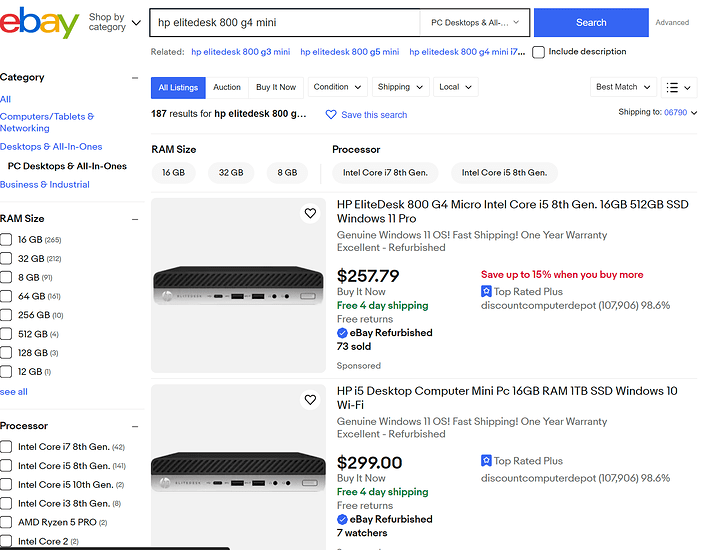The image represents a detailed view of an eBay search results page for "HP EliteDesk 800 G4 Mini." 

At the top, set against a white background, is the colorful eBay logo where each lowercase letter is uniquely colored: red 'e,' blue 'b,' yellow 'a,' and green 'y.' Below the logo is a functional search bar with the term "HP EliteDesk 800 G4 Mini" entered, alongside options to refine the search including "PC Desktops & All-in-Ones." The search button is blue with white text, and there's an "Advanced" search option.

On the left side, a menu labeled "Categories" features a drop-down allowing users to filter by "Computers, Tablets & Networking," "Desktops & All-in-Ones," and "Business & Industrial." Additional options refine the search further by RAM size or processor type.

Beneath the search bar, suggested related searches include "HP EliteDesk 800 G3 Mini," "HP EliteDesk 800 G5 Mini," and several configurations of the "HP EliteDesk 800 G4 Mini i7." Users can choose to include descriptions in their search using a checkbox labeled "Include Description." The page then displays "All Listings," distinguished by buttons for auction, "Buy It Now," condition (with a drop-down menu), shipping options, and local availability.

The search results show "187 results," with options to save the search. Filters allow users to narrow their choices by RAM size (8 GB, 16 GB, 32 GB) and processor type (Intel Core i7 8th Generation, Intel Core i5 8th Generation).

Finally, the image highlights two specific product listings with their respective prices and descriptions.